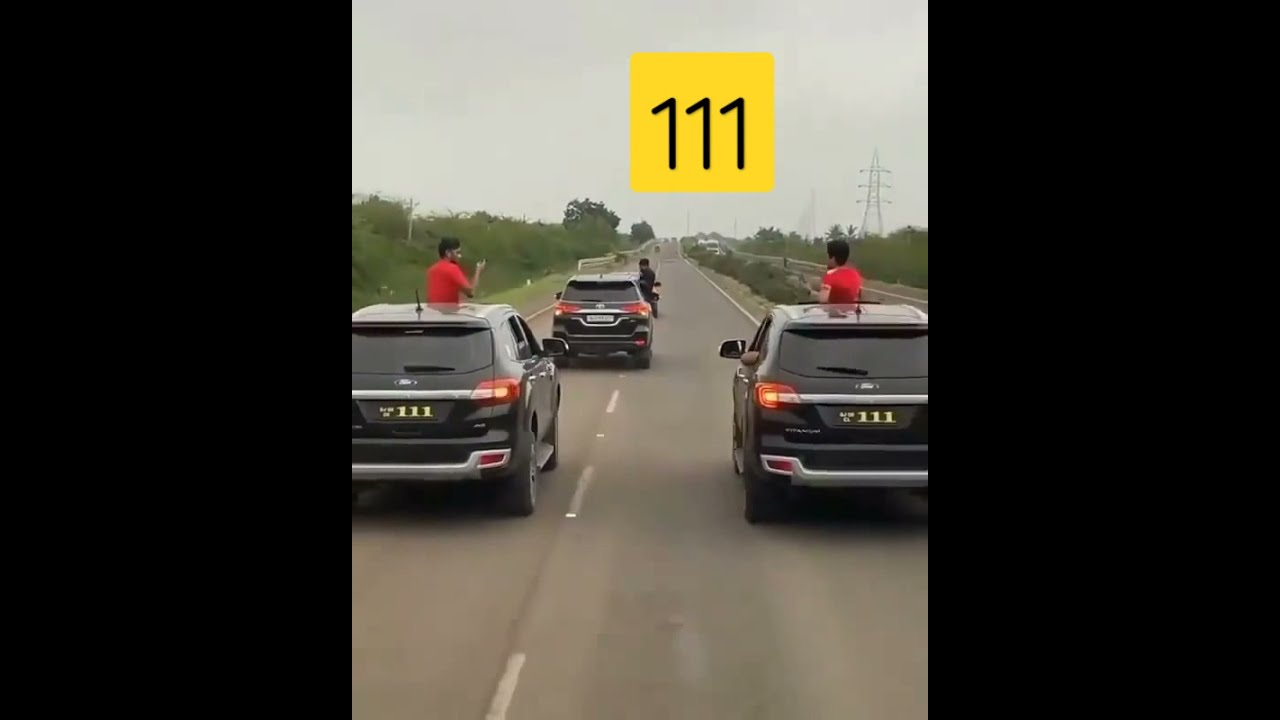The image depicts a cloudy day scene on a straight roadway flanked by greenery. On both sides of the road are lush green trees, with a secondary road separated by a strip of shrubs on the right. The primary road features three black SUVs, with the rear two positioned side by side and the lead SUV ahead, slightly straddling lanes. The SUV on the right is partially on the shoulder. The rear SUVs are Ford models, and the front one is a Toyota. All three vehicles carry passengers emerging from their sunroofs; the rear SUVs have occupants in red shirts, while the front SUV has an occupant in a black shirt. A notable detail includes matching yellow license plates on the rear Fords, each displaying the number "111". Additionally, a floating yellow sticky note effect with the number "111" is visible above the scene, suggesting it may be part of a video. Power lines and a tall power pole are visible in the background on the right, and the left side features grassy hills.